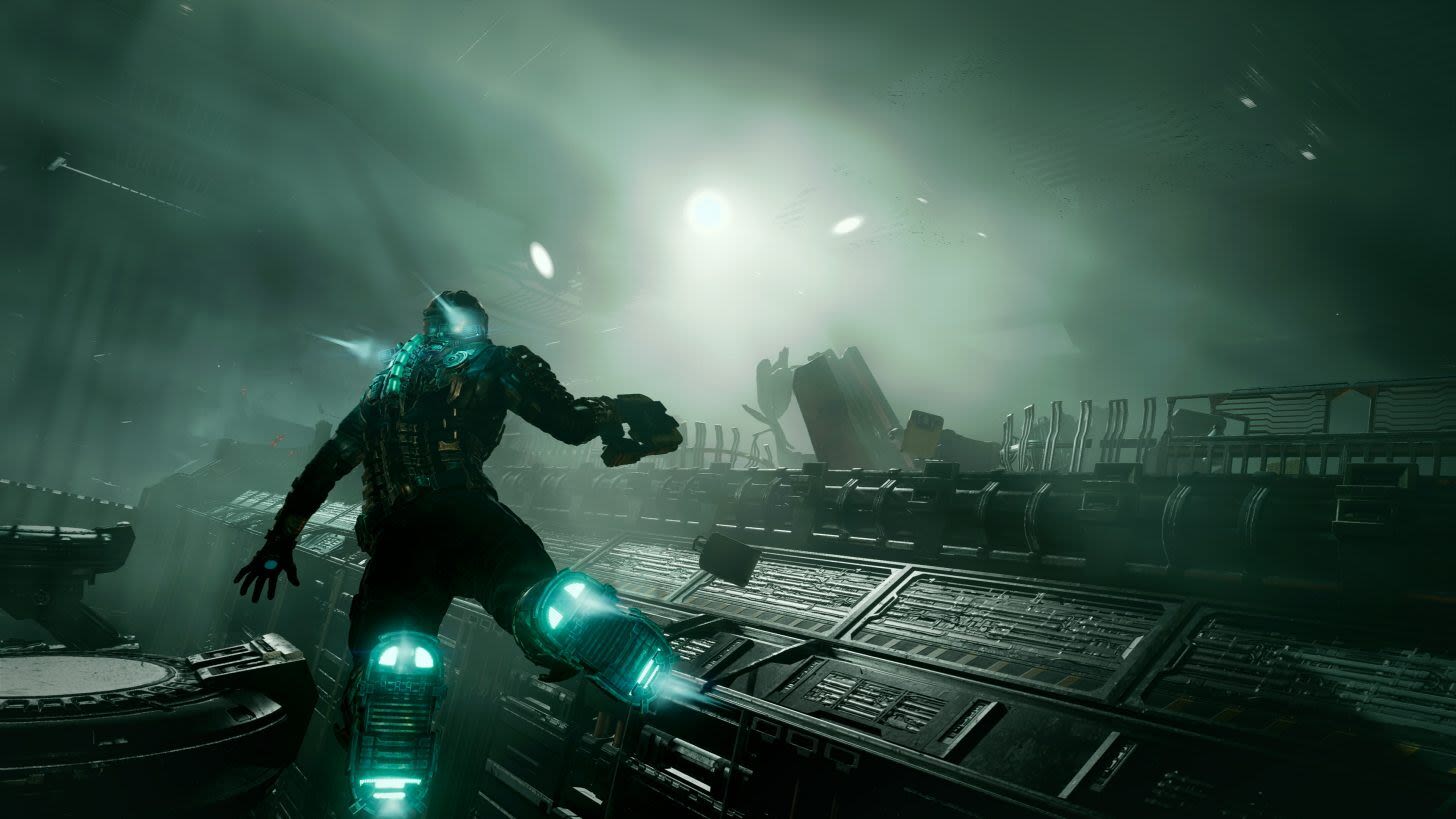The image is a screenshot from a video game, featuring a player dressed in a black suit equipped with a jetpack and jet boots emitting blue flames. The character, possibly robotic or wearing advanced futuristic gear, faces away from the camera, looking towards a distant, blinding light in the sky. The scene is set in a futuristic environment dominated by a very long metal building and multiple metal platforms to the left. The sky is cloudy and foggy, contributing to the dark and gloomy atmosphere of the image. The character’s suit has blue glowing elements, particularly around the head and knees, adding a vivid contrast to the predominantly gray and metallic surroundings. This image suggests a dynamic, possibly tense moment, with the character appearing ready to traverse the futuristic, fog-laden landscape.